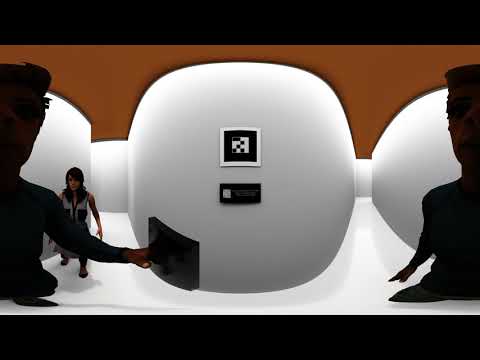The image showcases a futuristic, technologically-advanced scene centered around a large white, rounded rectangular pod. This central pod is connected to two other pods, creating a setup reminiscent of a space platform or some high-tech environment. The pod features a small picture, encased in a black frame within a white frame, and beneath it lies a black plaque with descriptive text that is not legible from this distance. 

Foreground elements include a male figure with a buzz cut who appears to be engaging with a lower compartment of the pod, possibly a small door or panel, suggesting interactivity or maintenance. To the left, a woman is walking towards the camera, adding a sense of movement and depth. Standing in what resembles a back room or maze-like structure is another man with a fresh haircut, who seems bewildered or confused. 

Overall, the composition blends clean, stark white tones with contrasting black elements, augmenting the space-like ambiance. An orange and black backdrop further enriches the scene, which seemingly depicts the group engrossed in some game or activity.